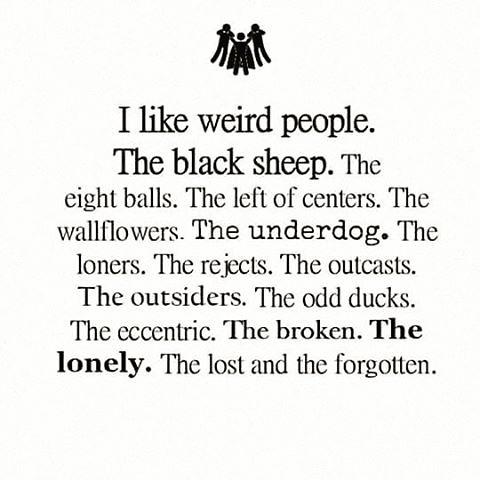The image features a quote on a white background, with black text in varying fonts and sizes. At the top of the image, a silhouetted figure, resembling a superhero with a cape, holds up two smaller silhouetted figures by the arms. Beneath this illustration, the text reads: "I like weird people. The black sheep. The eight balls, the left of centers, the wallflowers, the underdog, the loners, the rejects, the outcasts, the outsiders, the odd ducks, the eccentric, the broken, the lonely," with "the lonely" in bold. The quote continues in regular font: "the lost and the forgotten." The text lines are stacked vertically, with some phrases in bold for emphasis, creating a diverse and thought-provoking visual presentation.